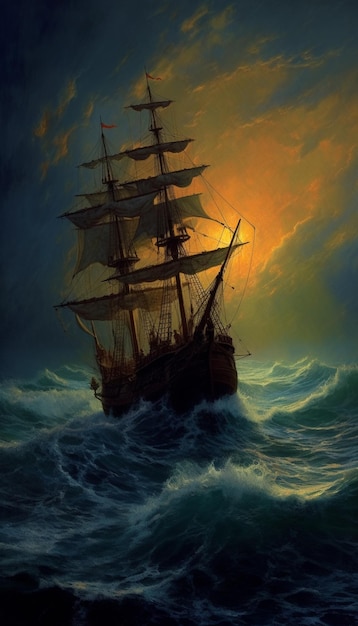This detailed painting, reminiscent of old-time maritime art, captures a large, old-fashioned pirate ship braving tumultuous, choppy waters with high, foamy whitecaps. The vessel, which evokes imagery of 16th and 17th-century explorers' ships, is tilted to the left, emphasizing the rough seas it battles. It sails under a sky dramatically split between stormy darkness and a brilliant, setting sun that breaks through the clouds, casting a stark, golden light directly behind the ship's central sail. The ship itself, adorned with multiple sails and two prominent red flags, is manned by numerous sailors. The water below is a mix of dark and light blue hues, accentuated by white spray, while the sky is a blend of dark blue, stormy clouds and vivid streaks of yellow, orange, and red, creating a striking and rugged seascape.